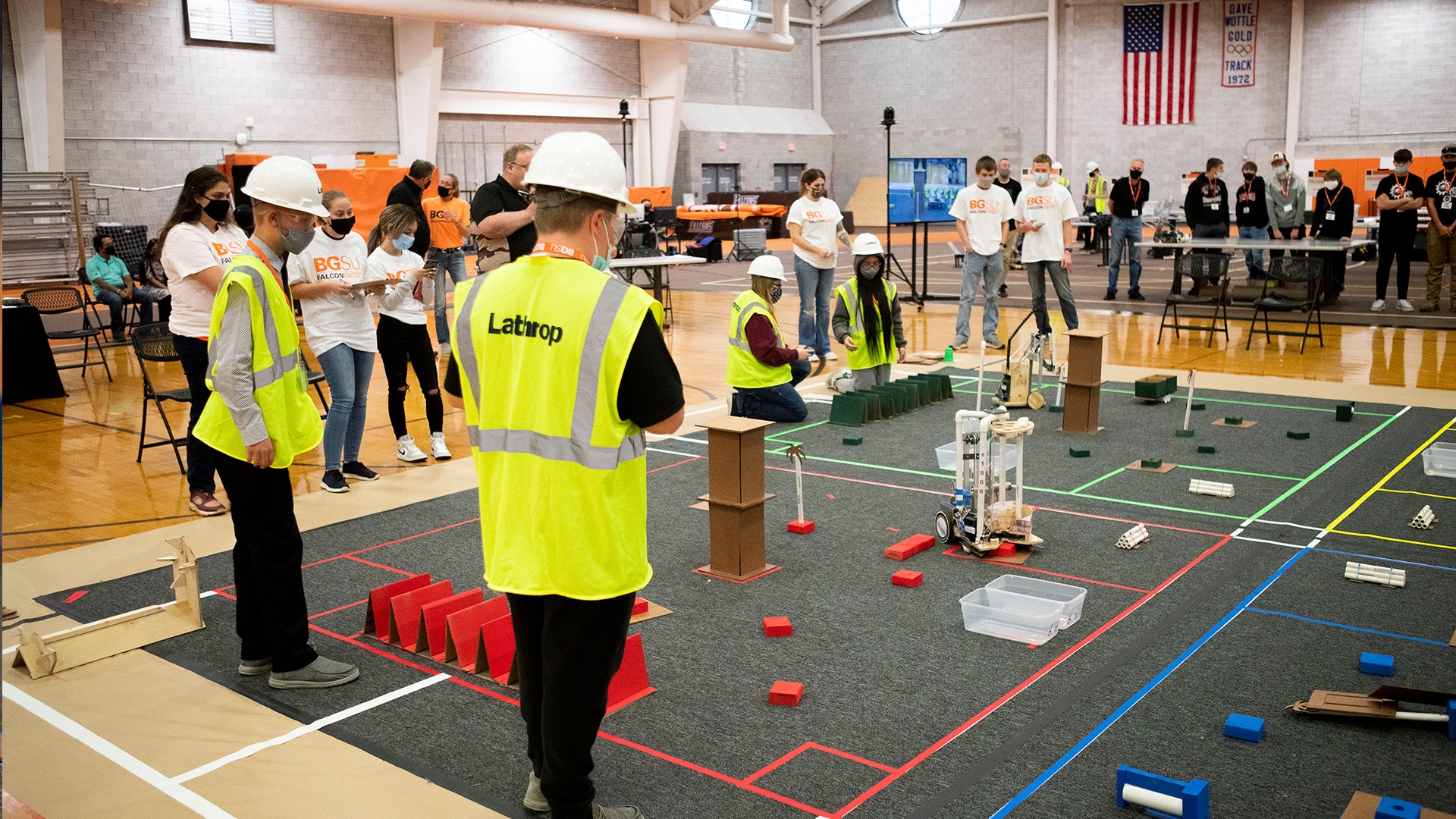In this detailed photograph taken inside a large gymnasium, we see a dynamic scene centered around what appears to be an intricate engineering competition or safety demonstration. The gymnasium floor is predominantly covered in a large gray carpet, with specific areas divided by green and red colors, indicating where different teams are stationed—two individuals on the green side and two on the red side. Each participant is equipped with safety gear, including white helmets, green safety vests with a gray stripe, and standard work attire.

Surrounding the main activity, a sizable audience is gathered, consisting of people dressed in causal attire. Among them are some individuals wearing white shirts with visible writing and others in darker shirts seated at a table, many adorned with lanyards. The overall scene is well-organized with a considerable amount of focus directed towards the central area where there's a large device featuring wheels and plastic components, suggesting a demonstration or experiment involving engineering principles, possibly even involving toy-like blocks referred to as blue, red, green, and yellow blocks.

The gymnasium itself is characterized by white and greyish brick walls, a large TV screen, and prominently, an American flag hanging on the far wall. The setting is a lively mix of concentrated activity and engaged onlookers, creating a robust atmosphere of community and shared interest in the proceedings.